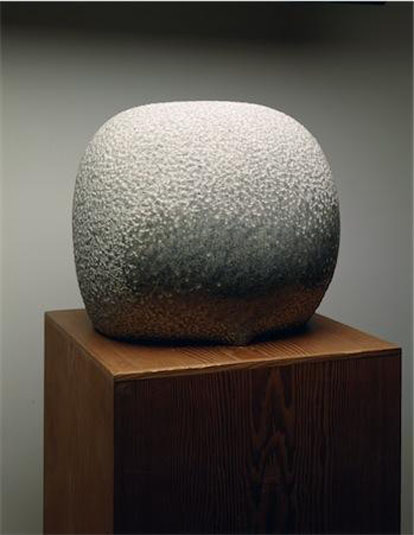This photograph features a striking piece of modern art, capturing a large, almost spherical sculpture that resembles a marshmallow or boulder, encased in shades of gray with a rough, mottled texture on the top and left parts. The sculpture, which seems larger than a watermelon, rests prominently on a finely-grained, brown wooden stand with visible corners facing the viewer. The backdrop is a gradient wall, transitioning from light gray at the top to black near the bottom, suggesting a light source casting illumination from above. The composition is solely focused on this singular abstract object, devoid of any text, signatures, or other items, emphasizing the contrast between the smooth wood and the rough, gray sculpture.